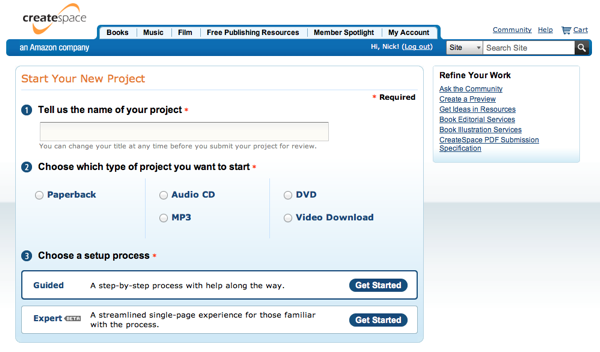This screenshot showcases a webpage from the retro-styled CreateSpace website, which appears outdated. CreateSpace is prominently displayed in the upper left corner with the word "Create" in bold, accompanied by a yellow swirl around it. Directly below is a blue banner stating "an Amazon company," indicating that CreateSpace is an Amazon subsidiary. On the right side of this blue banner, the user’s name is shown with a greeting, "Hi Nick!" next to a logout button and a site search bar.

Occupying the majority of the screenshot is a light-colored background form area. At the top, in bold orange text, it reads "Start your new project." The section below is divided into three steps: 

1. In a circled number '1', it prompts users to "Tell us the name of your project," accompanied by a text box for input.
2. Number '2' instructs users to "Choose which type of product you want to start," offering clickable options such as paperback, audio CD, MP3, DVD, or video download.
3. Lastly, number '3' asks users to "Choose a setup process," providing options for either a guided setup or an expert setup.

The overall design has a distinctly nostalgic, retro feel typical of early 2000s web aesthetics.